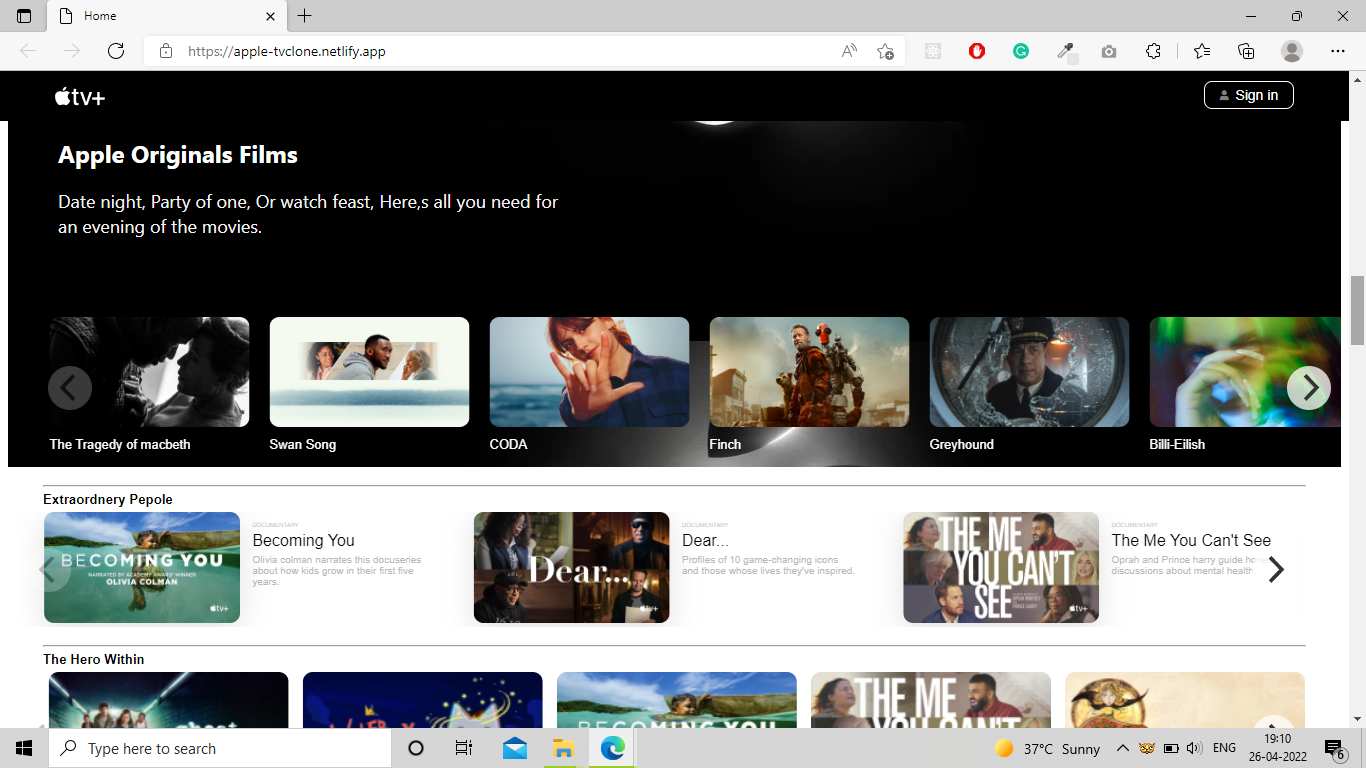Screenshot of the Apple TV Website:

At the top of the screenshot, there is a gray banner with a square box and the active "Home" tab highlighted in white. To the right of the "Home" tab, the banner contains a plus sign, a minus sign, a copy icon, and an 'X' for closing the page.

Immediately below the gray banner on the left-hand side, there are two light gray arrows; one points to the left and the other to the right. Next to these arrows is a circular arrow icon used for refreshing the page. The address bar displays "https://apple-tvclone.netify.app" with a padlock icon indicating a secure connection. The bar also features a red octagon with a white hand inside, a green circle with an arrow resembling a 'G,' an eyedropper icon, a camera icon, a puzzle piece icon, a star icon, a plus icon, a user ID icon, and three vertical dots.

The main section of the webpage contains a prominent black rectangular box. At the top of this box is the Apple TV+ logo, with the Apple icon followed by "TV+." Below the logo, the text reads "Apple Original Films." Further down, a line of text states: "Date Night, Party of One or Watch Feast. Here's all you need for an evening of movies."

Beneath this, there's a horizontal stream of movie thumbnails showcasing titles such as "The Tragedy of Macbeth," "Swan Song," "CODA," "Finch," "Greyhound," and "Billie Eilish." Underneath the stream of movie images is another banner with the title "Extraordinary People," and although 'Extraordinary' is misspelled in dark letters, it lists movies like "Becoming You," "Dear," and "The Me You Can't See."